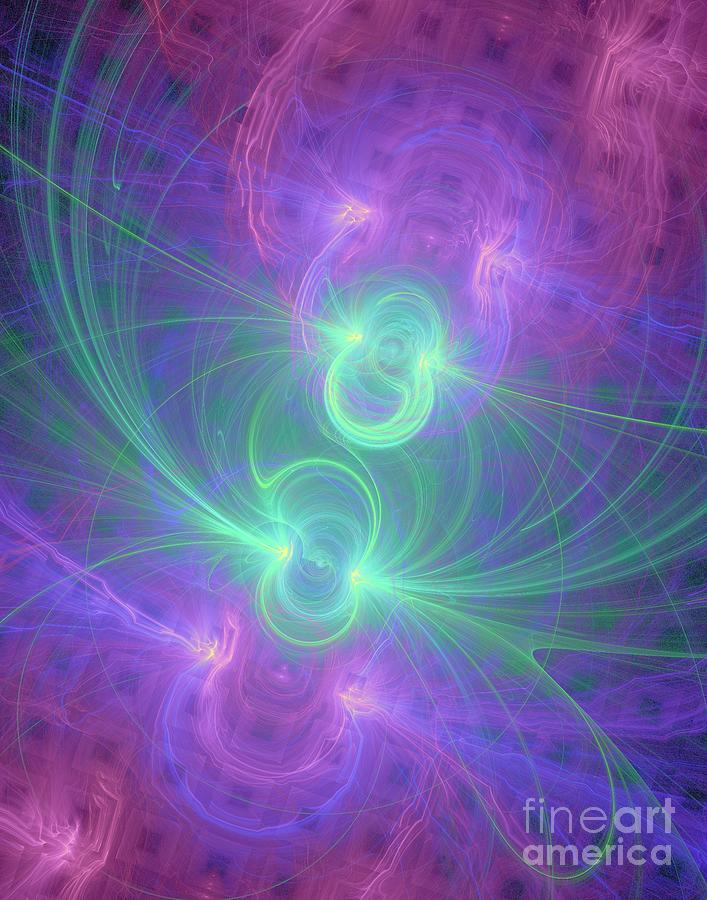This vivid, abstract digital artwork by Fine Art America showcases a dynamic array of neon colors and intricate patterns. Dominated by hues of neon green, purple, pink, yellow, and white, the composition features multiple pulsating circles set diagonally from the center, giving the impression of a constant, vibrant movement. The top two neon circles radiate in lime green, while the bottom circles transition into a mesmerizing blend of blue and purple. The background resembles a textured fabric print with small, white squares that have dark centers, reminiscent of a waffle pattern. These squares are interspersed with fine, lightning-like electrical currents in pink, adding to the laser-like effect. The circles themselves loop repeatedly, forming shapes akin to a figure-eight, with flares that resemble wings. All these elements converge towards the center, creating an impression of illuminated waves. The artwork’s sophisticated neon bands and radiant figures make for a compelling visual spectacle. In the bottom right corner, a semi-transparent watermark in 50% white reads "Fine Art America," further authenticating the piece as a remarkable example of computer-generated fine art.